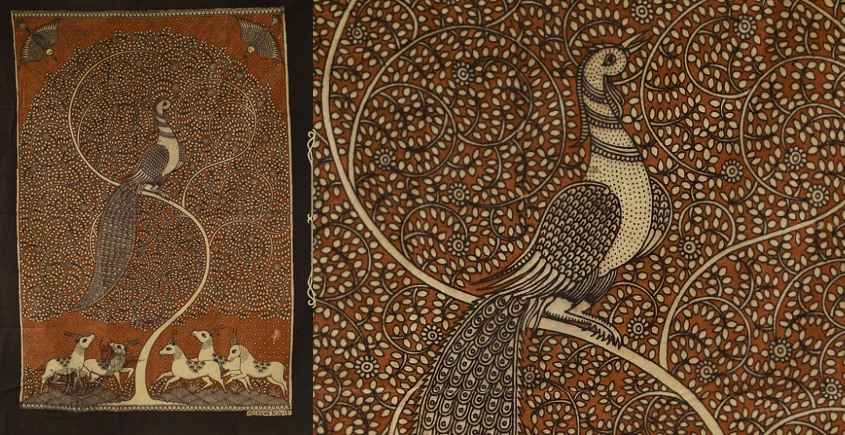The image displays a highly detailed art piece of a peacock, captured in a landscape orientation. On the left third of the frame, the entire fabric piece is visible, while the right two-thirds offer a zoomed-in view of the peacock itself. The artwork, resembling a fabric or rug, features intricate details: the peacock is centered, perched on a bare tree branch with its tail feathers potentially doubling as leaves. The background contrasts dark maroon-red hues with foreground colors of yellow, white, dark brown, and cream. Surrounding the peacock is a patterned array of curving leaves and vines that form a tree. Below the branches, several animals resembling horses or deer with two long horns gaze upward at the exotic bird. Additionally, two birds can be seen diving towards the peacock from the top corners of the image. The piece is framed in a black border, enhancing the rich, intricate details of this stylized depiction. The peacock itself, with its beak open and looking upwards, showcases an abundance of feathers and vibrant patterns, making it the focal point of this elaborate and colorful artwork.